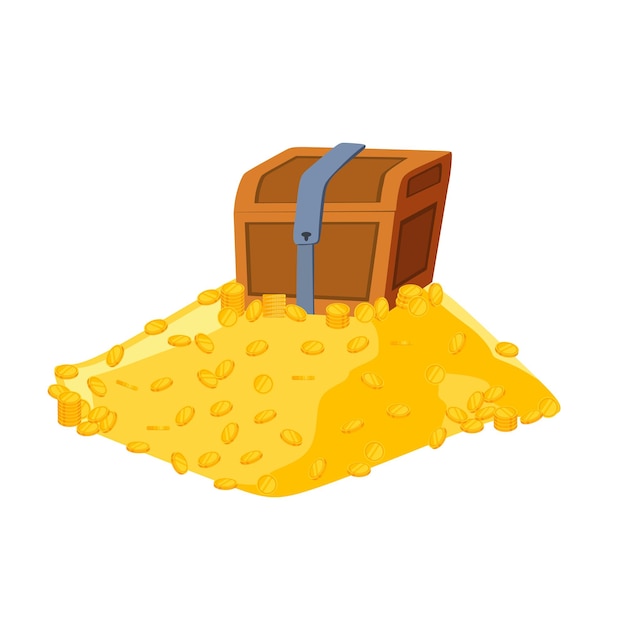The image is a simple, stylized illustration set against a plain white background with no border or additional text. At the center, a small, pirate-like treasure chest is depicted. The chest is made of wood, characterized by various tones of brown, and features darker brown panels on the sides and front. It is secured with a distinctive, gray metal strap across its middle that includes a keyhole shaped like a skeleton head. 

This small chest sits atop a thick, uneven pile of gold coins that vary in shades of gold, from a yellow hue to a more subdued brownish gold. The pile is denser and slightly elongated on the left side. Individual coins and stacks can be discerned around the edges and across the mound, enhancing the impression of a treasure trove. The overall impression is of a digital, cartoon-like image of a treasure chest surrounded by a substantial amount of gold coins, all set on a stark white backdrop.